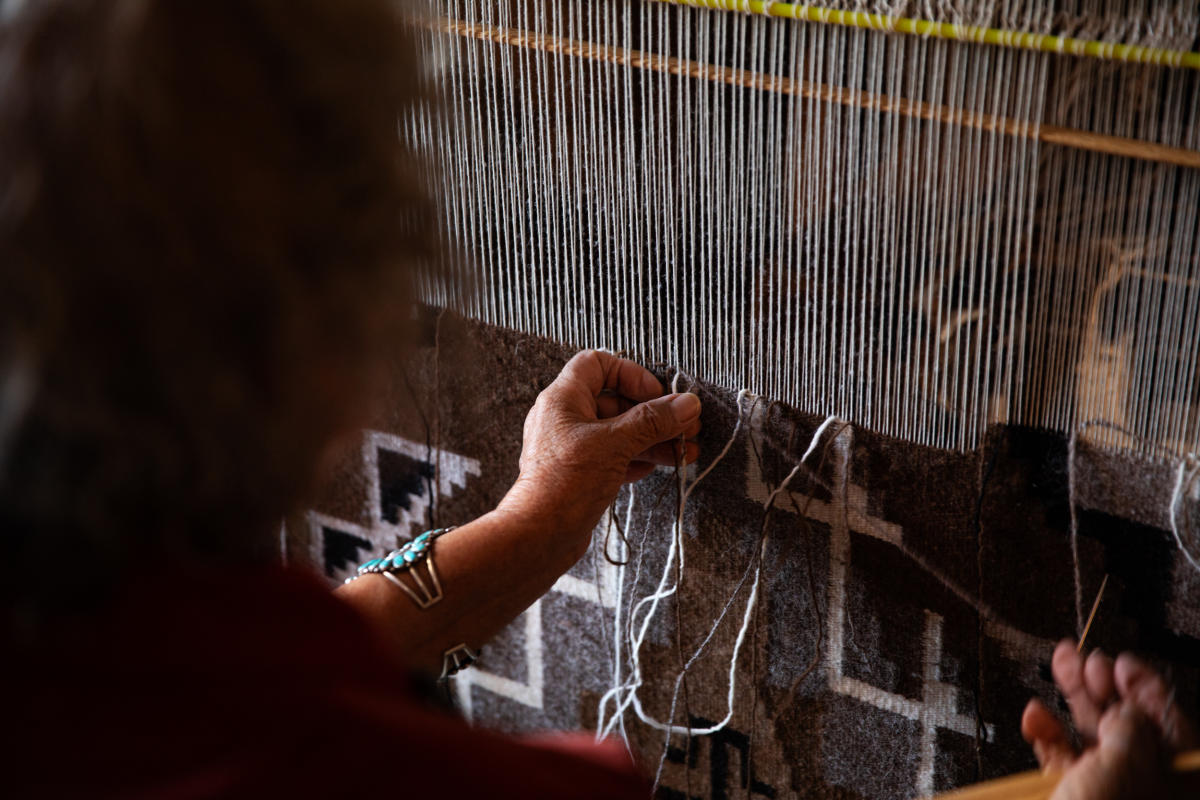In this detailed photograph, an older person with shaggy gray hair and wearing a red shirt is intricately weaving on a loom. The image is taken from over their shoulder, focusing on their wrinkled hands expertly maneuvering the needle and threads to create a geometric pattern. The loom features vertical strings stretching from top to bottom, with many loose threads that the person works into the fabric. The emerging pattern, which might be part of a traditional Americana blanket or rug, predominantly features shades of tan and off-white. The top half of the photo showcases the unfinished cloth with exposed strings. The individual sports an interesting turquoise bracelet on their left wrist. Their face is not visible, emphasizing the meticulous work of their hands in this engaging and detailed composition.